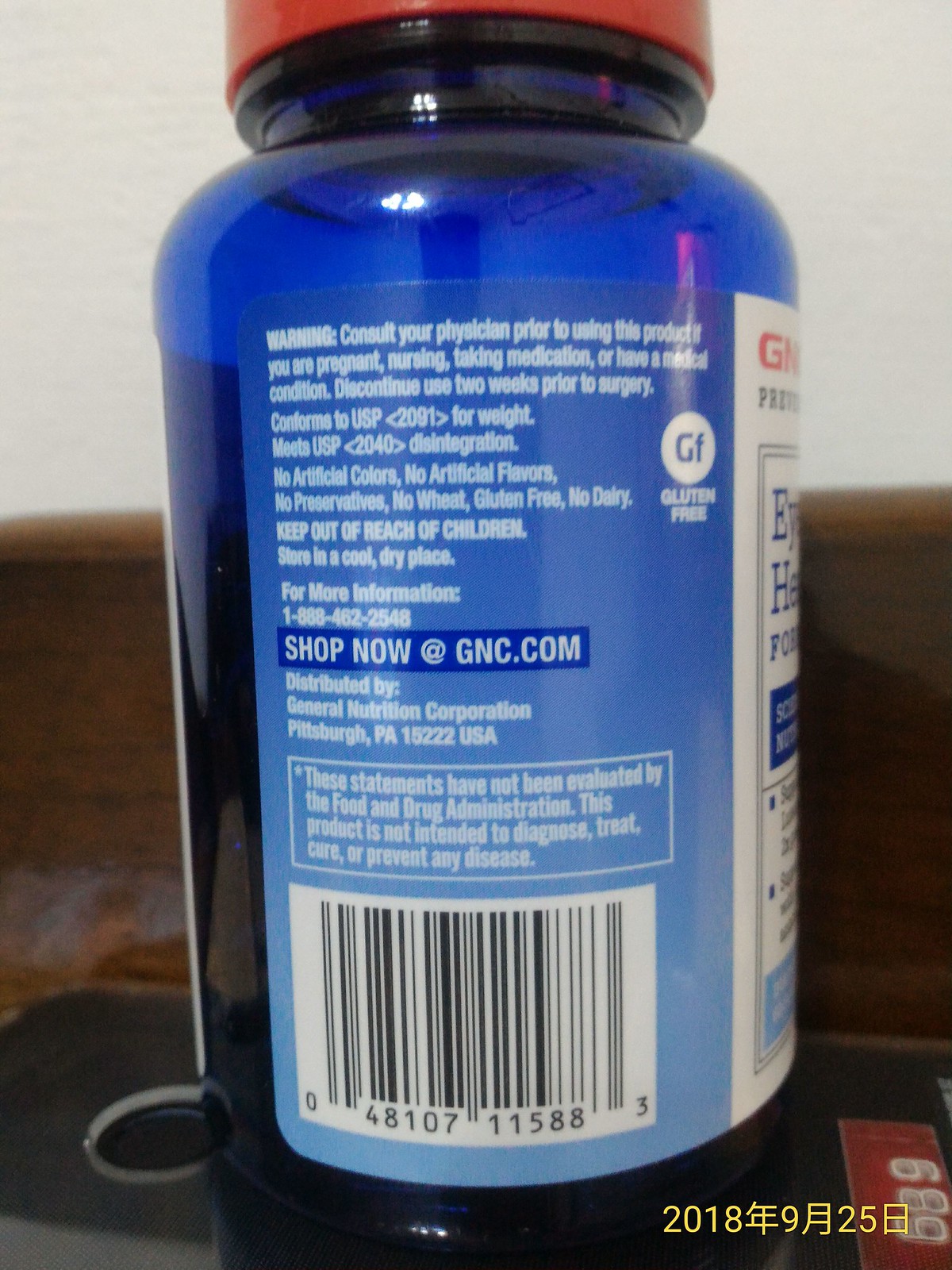This extreme close-up photograph captures a scene on a brown wooden table surface with a white wall in the background. In the corner of the image, there is a date stamp featuring Asian text, indicating the date as 2018-09-25. On the table sits a black cell phone, and resting on top of it is a transparent blue medicine bottle with a dark liquid inside and topped with a red cap. The back of the bottle is prominently visible, displaying various warnings and product information. The label, primarily blue and white, includes a banner that reads "shop now at GNC.com" and features additional details such as "no artificial colors, no artificial flavors, no preservatives, no wheat, gluten-free, dairy-free, keep out of reach of children, store in a cool, dry place." It also carries the message to consult a physician before use if one has medical conditions or is taking medication. The barcode and distribution information by General Nutrition Corporation in Pittsburgh, PA, USA, are also visible. The text advises discontinuing use two weeks prior to surgery, notes product compliance with USP 2091 and 2040 standards, and mentions that the statements have not been evaluated by the FDA.